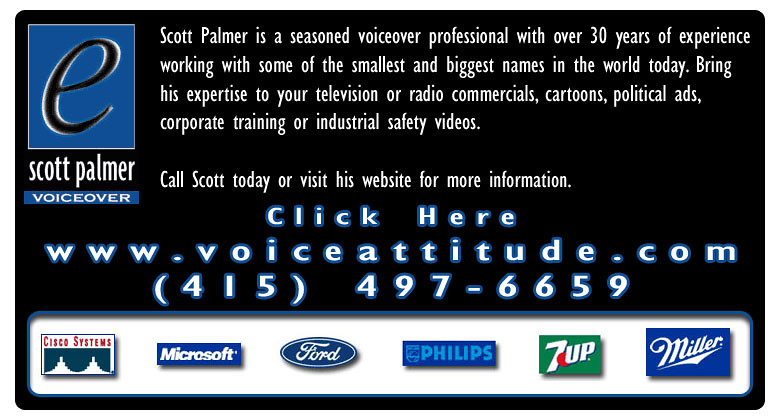The image depicts an internet advertisement styled like a business card for Scott Palmer, a seasoned voice-over professional with over 30 years of experience. The webpage features a black background with white lettering. In the upper left corner, there is a logo with a black 'E' on a blue background inside a white-bordered square. Below the logo, "Scott Palmer Voiceover" is prominently displayed in white text. On the upper right side, the white text elaborates on Scott Palmer's extensive experience and qualifications, highlighting his work with a diverse range of clients from well-known brands to smaller companies. It mentions his services for television and radio commercials, cartoons, political ads, corporate training, and industrial safety videos. A call to action follows, encouraging viewers to contact Scott via phone or visit his website for more information. Below this text is a blue-bordered white button labeled "Click Here," along with Scott's website, www.voiceattitude.com, and phone number, 415-497-6659. At the bottom, a white bar displays logos of various companies Scott has worked with, listed from left to right: Cisco, Microsoft, Ford, Philips, 7-Up, and Miller.